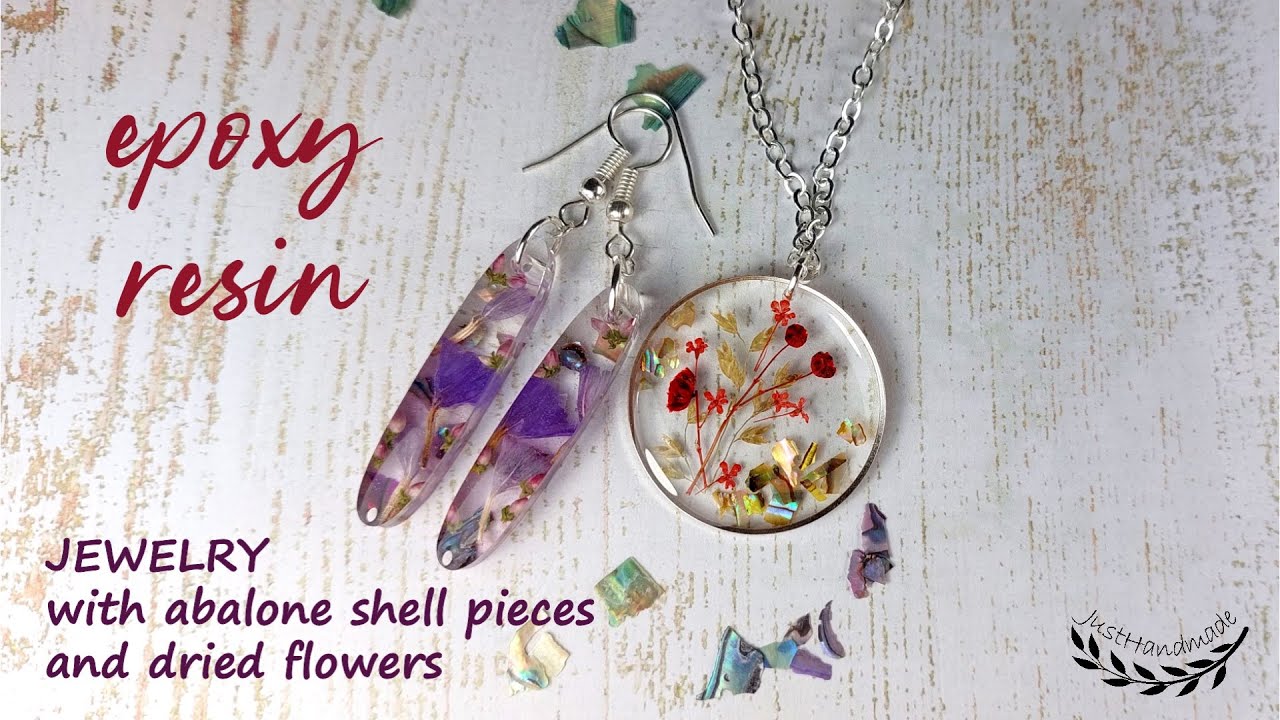This photograph features an advertisement for "Just Handmade" jewelry, prominently displayed on a distressed, white-painted wooden table that reveals the grain beneath. The image showcases a necklace and a pair of dangle earrings, meticulously crafted from clear epoxy resin embedded with abalone shell pieces and dried flowers. The earrings, with silver clasps, are elongated, approximately two inches long, featuring a mix of embedded materials predominated by purple hues, along with accents of red, blue, tan, and turquoise. The necklace is a silver chain with a circular epoxy resin pendant, containing small, red and yellow dried flowers, and multicolored shell pieces. The background includes a vertical streaked pattern of white, brown, and red, with red and purple script in the upper left and lower left corners reading "Epoxy Resin" and "Jewelry with Abalone Shell Pieces and Dried Flowers," respectively. The bottom right corner displays the "Just Handmade" logo, emphasizing the brand's artisanal focus.